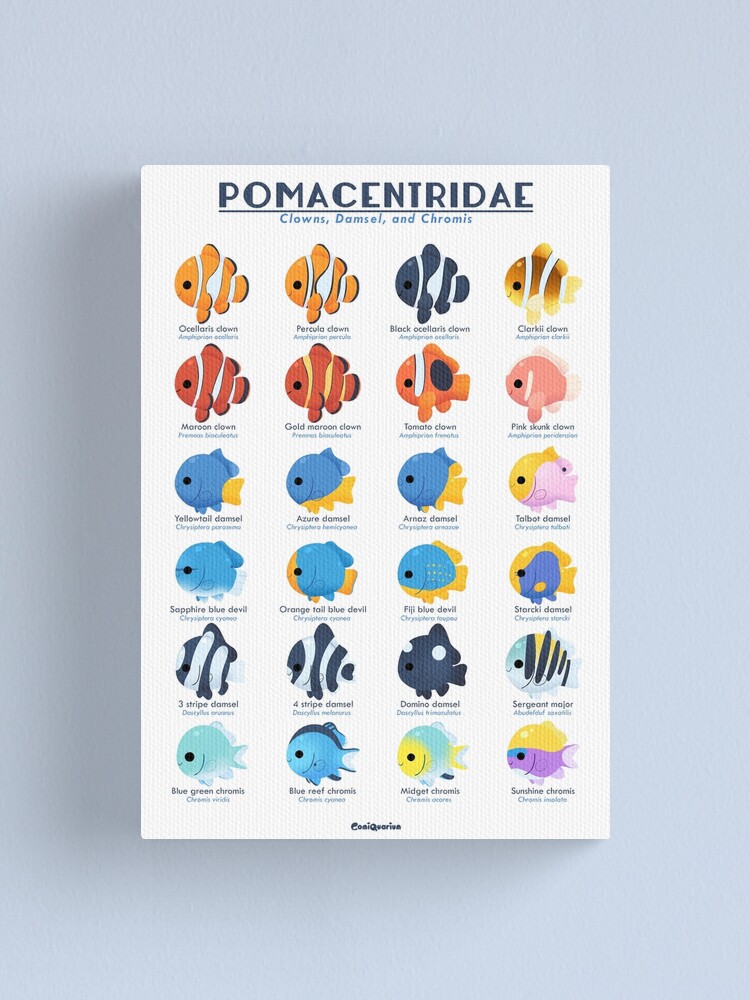This is a detailed color photograph of an informational poster serving as an identification guide for tropical fishes. The white poster is set against a baby blue background. At the top, in bold black lettering, it reads "POMACENTRIDAE," with a line underneath. Below this, in blue text, are the words "Clowns, Damsels, and Chromis." The poster features six rows, each containing illustrations of four different fish, making a total of 24 fish. 

The fishes are depicted in vibrant, cartoonish patterns rather than realistic images. In the first row, there are two orange and white clownfish, a black and white clownfish, and a brown and white fish. The second row includes a red and white fish, a red and orange fish, an orange fish, and a pink fish. The third row showcases a blue fish with a yellow tail, another blue fish with a yellow belly and tail, a blue fish that has a half-yellow body, and a fish with a yellow head and a pink body. The fourth row features blue and white fish, blue and yellow fish, black and white fish, and a black and white spotted fish. The fifth row includes a fish that is blue, yellow, and black. Finally, the bottom row presents a light blue fish, a light blue and yellow fish, a yellow fish, and a purple fish.

Overall, the poster provides a neat and colorful depiction of various fish species, enabling easy identification with a clean, organized layout on a shiny light blue background.